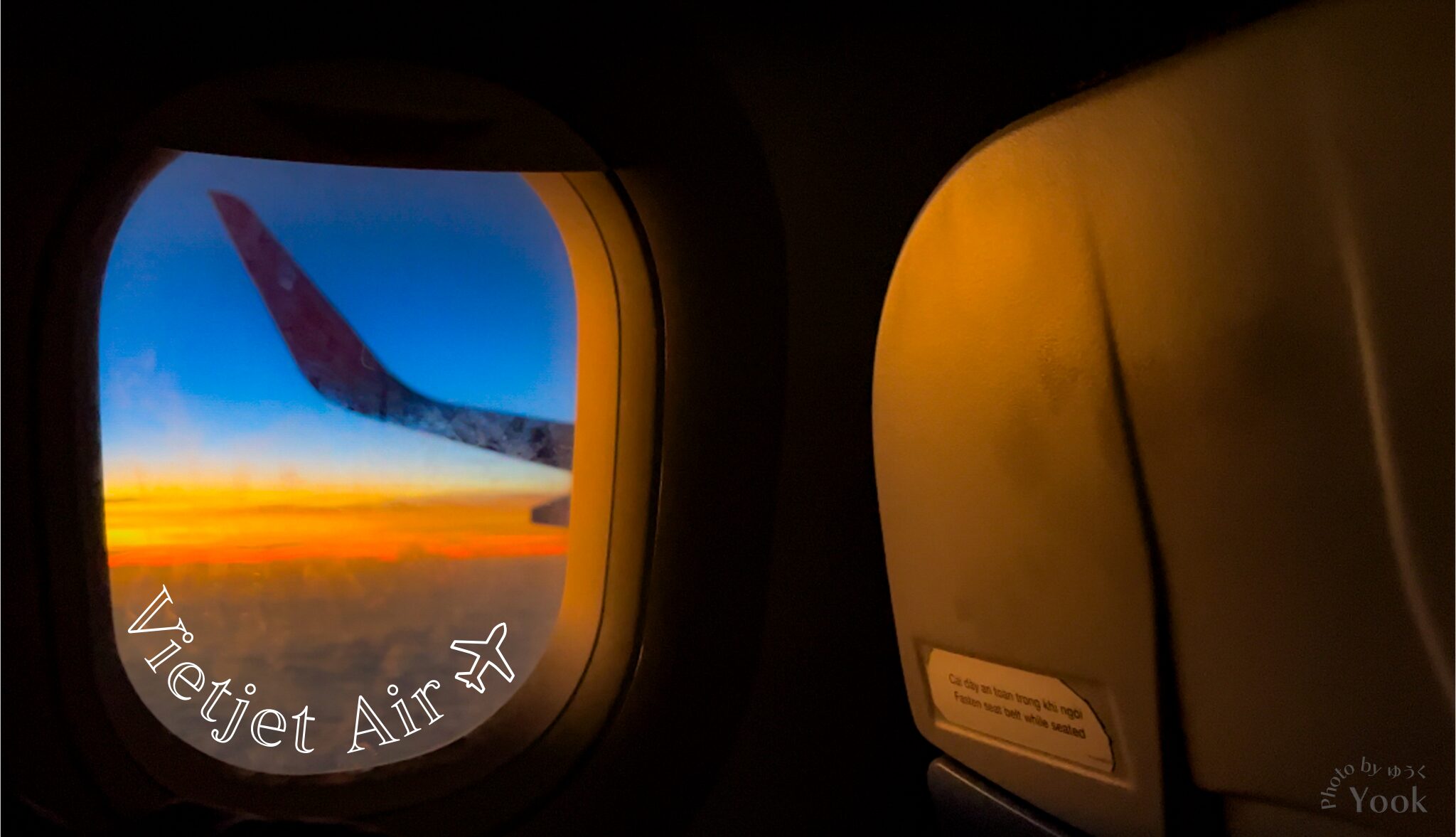This photograph is taken from inside a passenger airplane during sunset or sunrise, viewed from a window seat. The scene captures a vivid gradient sky transitioning from deep blue at the top to warm orange, yellow, and red hues near the horizon. The sunlight casts a cozy orange hue on the back of the seat in front of the photographer, creating a warm and inviting atmosphere. On the right side of the image, part of the upper back of the next row's seat is visible, while on the left, the plane's oval-shaped window frames the outside view. Through the window, the hazy outlines of distant land and the tail wing of another plane are discernible. Across the bottom of the window, in a semicircle, are the words "Viet Jet Air" accompanied by a small airplane icon. The image has a dark overall tone, except for the sunlit areas and text in the lower right corner that reads "Photo by Yook."